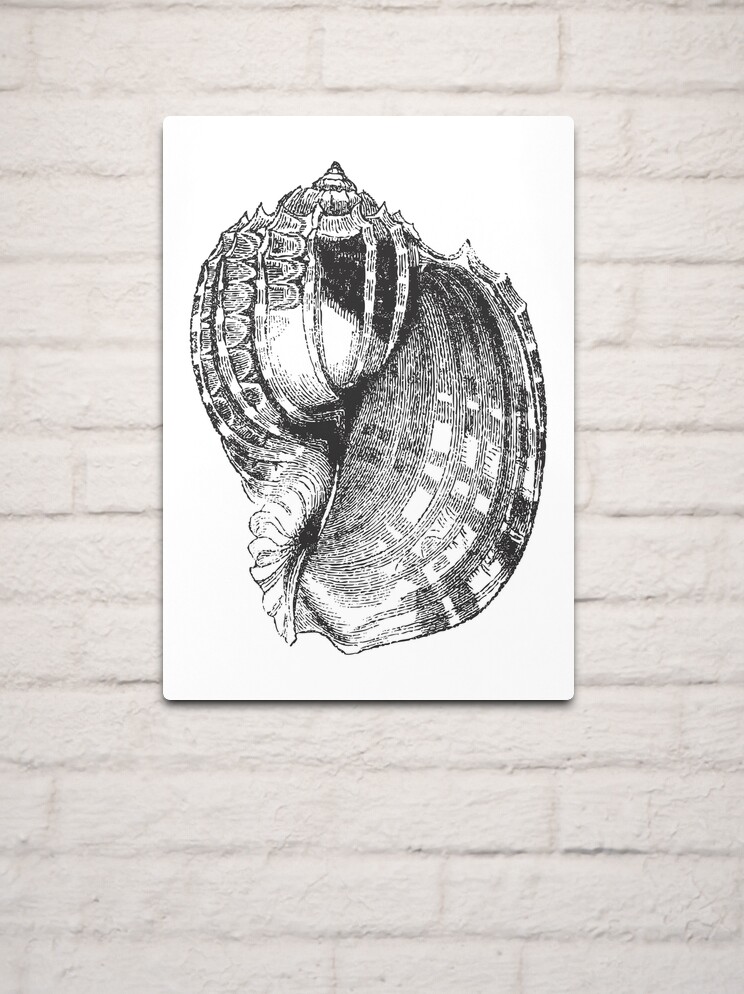The image is a photograph of a black and white illustration of a conch shell on a white brick wall. The wall has been heavily painted, leaving only faint outlines of the bricks and mortar visible. The illustration itself is on a rectangular white background, possibly a piece of metal or board with a whitish silver finish, as it is not framed. The conch shell dominates the entire page, with the large open side to the right and the narrow, pointed end at the top left. The shell features distinctive stripes and striations, giving it a textured appearance. The overall shape of the shell curves like a large 'C' on the left, with the body portion extending to the right.